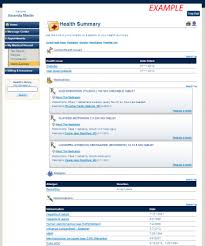This is a detailed caption for the image provided:

---

**Detailed Description of a Health Summary Page Screenshot:**

The image depicts a vertical, rectangular screenshot of a health summary page. At the top of the page, there is a dark horizontal banner that slightly extends down the left and right edges, giving the top a bordered look. The background beneath this banner is white. In the upper right-hand corner of the page, the text "Example" is prominently displayed in red. Positioned towards the center left, the document title "Health Summary" is clearly visible.

Beneath this title, an icon resembling a folder with a red cross in its center is present, symbolizing medical records or health information. A vertical menu box is aligned to the left side of the page, aiding in navigation. On the right side, the page features numerous lines of text, mostly rendered in blue, though the specifics are not legible. The various sections of text are distinctly separated by wide, dark blue horizontal borders, enhancing readability and section demarcation.